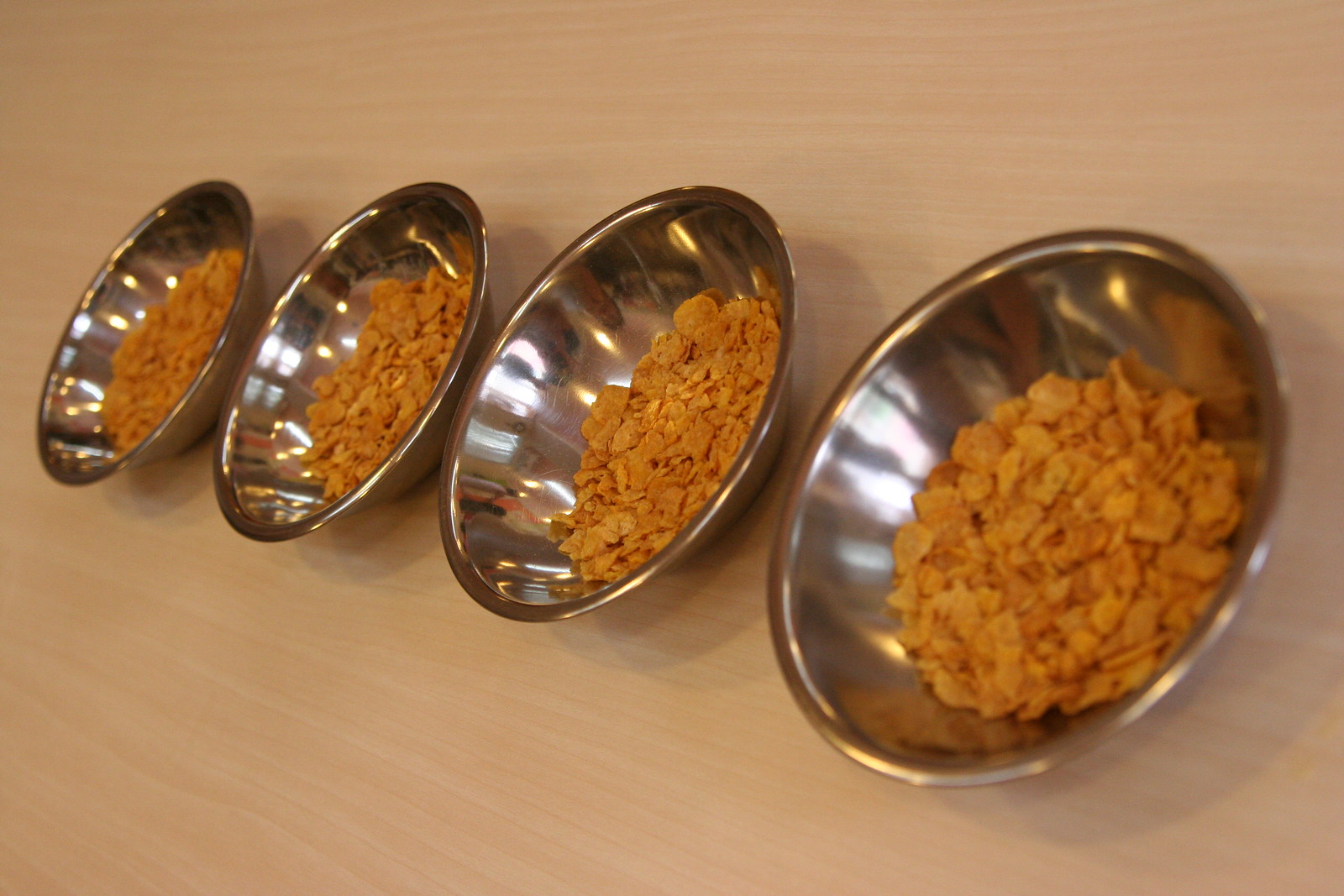This photograph captures a simple yet intriguing scene of four shiny, silver metal bowls lined up on a blonde wooden surface, likely a kitchen counter or table. These metal bowls, which bear a striking resemblance to either mixing or dog dishes, are illuminated by a light source positioned behind the camera, casting distinct shadows on the wood below. Each bowl is filled with golden-brown cornflakes, enhancing the reflective quality of the metal and accentuating the toasted color of the cereal. The bowls are arranged from a closer perspective in the lower right, receding to the upper left, and are slightly tilted upwards, giving the impression of being wall-mounted. The image is horizontal with no text or lettering, focusing solely on the interplay of light, texture, and the simplicity of the everyday items depicted.